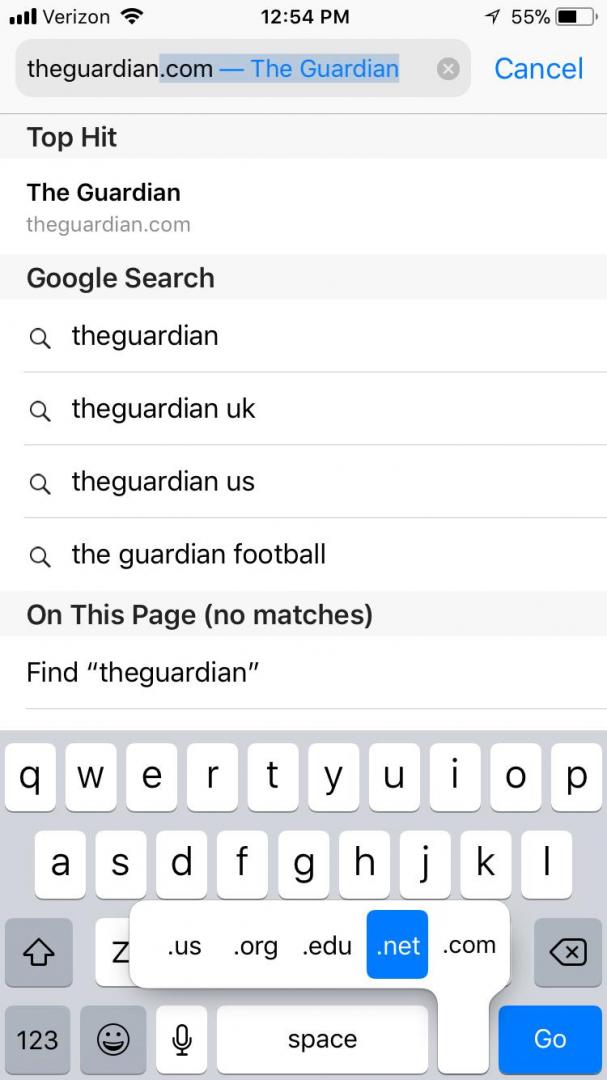This rectangular, vertically-oriented image appears to be a screenshot taken from a cell phone. At the very top, a grayish border banner spans across the image. The left side of this banner displays a cell phone signal with four out of four bars, the word "Verizon," and a Wi-Fi signal showing full strength. Centrally positioned is the time "12:54 p.m." On the right side of the banner, there's an upward-pointing arrow next to the number "55%" and a battery icon indicating it's about halfway charged.

Beneath this, within the same gray banner but in a darker shade, there's an oblong box containing the text "theguardian.com - The Guardian," with an "X" to the right, and on its right side, the word "Cancel" in blue text. Following this is a thin gray bar displaying "Top Hit" in black text.

Lower in the image, a white box repeats "theguardian theguardian.com," followed by another light gray box labeled "Google search." Down the left side of the screen are search symbols, with respective text next to them featuring variations of "theguardian," including "theguardian," "theguardianspaceuk," "theguardianspaceus," and "theguardianfootball."